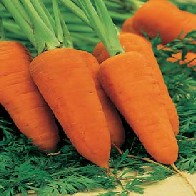This is a square close-up photograph of a cluster of six very large and seemingly perfect bright orange carrots, laying at a 45-degree angle on a possibly artificial grassy or leafy green surface. The carrots, fatter than typical, have vibrant, detailed, and leafy green tops, with the tips of their roots visible. Their striking uniformity in color and smooth appearance might make them seem almost unreal or artistic renderings. Scattered around and intertwined with the primary carrots are a few more in the background, all aligned towards the left side of the image. The setting and presentation of the carrots lend an impression of them being part of an artistic or staged scene, despite their realistic detailing.